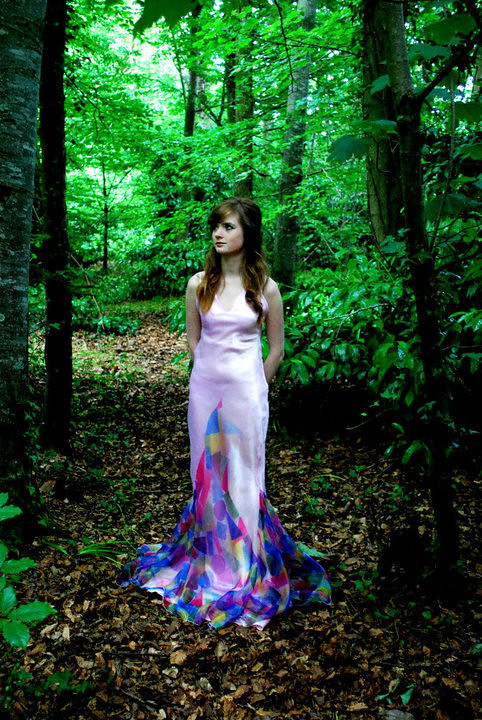This is a vertically aligned rectangular image of a young girl standing in a vibrant forest setting. She appears to be in high school, possibly dressed for prom in a stunning gown. The girl, who has long wavy brown hair cascading over her shoulders, is striking a pose with her arms behind her back, facing the viewer but gazing off to the left. Her dress features a sleeveless bodice with a plunging neckline and is primarily white or light pink at the top. Below the waist, the gown flows into a captivating array of geometric shapes in various colors, including blue, yellow, pink, purple, and green. She stands on a pathway covered in brown mulch or leaves, surrounded by tall, narrow tree trunks with green foliage. The scene is bathed in daylight, with patches of sky visible through the tree branches at the top of the image, adding to the enchanting woodland atmosphere.